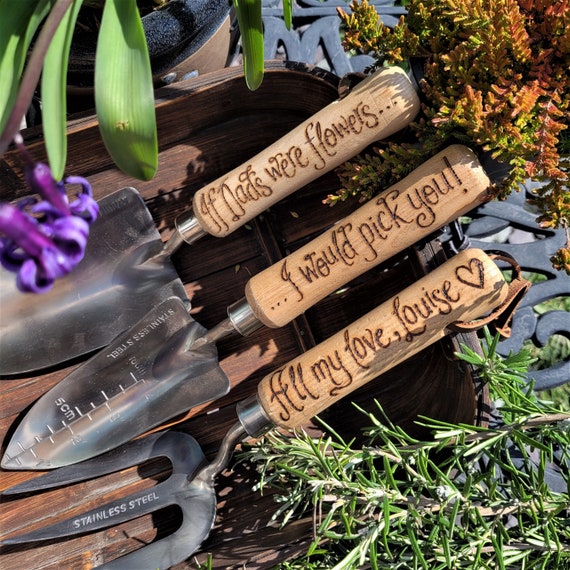This detailed photograph features a close-up of three personalized gardening tools—a trowel, a spade, and a three-pronged fork—each with wooden handles and metal heads. The handles are intricately engraved with messages: the top one reads, "If dads were flowers...," the middle one says, "I would pick you," and the bottom one says, "All my love, Luis," accompanied by a heart. These tools rest on a wooden tray, which is set against a backdrop of various plants and foliage. The top left of the image shows banana leaves, while the top right features greenish-orange leaves from another plant. In the bottom right corner, some rosemary and purple flowers are visible, adding a touch of color. A wrought iron design in the background suggests that the arrangement is placed on an outdoor table, creating a charming and warm scene.